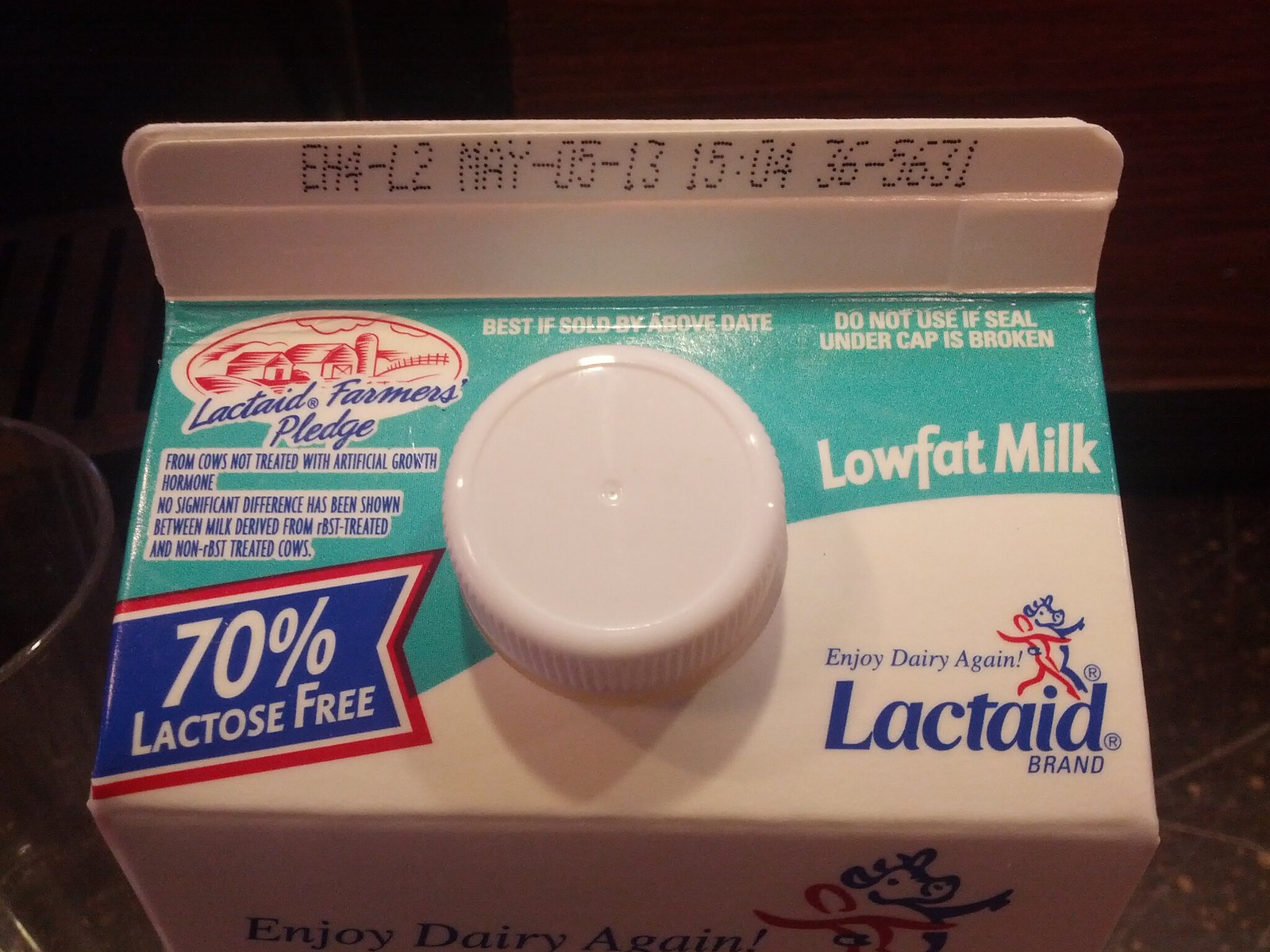This image showcases a close-up of the top of a low-fat carton of Lactaid brand milk, highlighted by its white base color and a green fan pattern on the screw-on white lid. Prominently featured is text that reads "EH4-L2MAY-05-13-15-04-36-5631" which appears to be a code or expiration date. The silhouette of a traditional farm scene, including a barn and silo, is displayed in red on the top corner, accompanied by the label "Lactaid Farmers Pledge." Another significant detail is the claim "from cows not treated with artificial growth hormones," followed by a note stating no significant difference has been indicated between milk from RBST-treated and non-RBST-treated cows. In the lower right corner, a blue-flag graphic, bordered in red and white, prominently states "70% lactose free." Additional text across the carton includes "Enjoy Dairy Again," emphasizing the Lactaid brand's commitment to providing dairy products suitable for those with lactose intolerance.